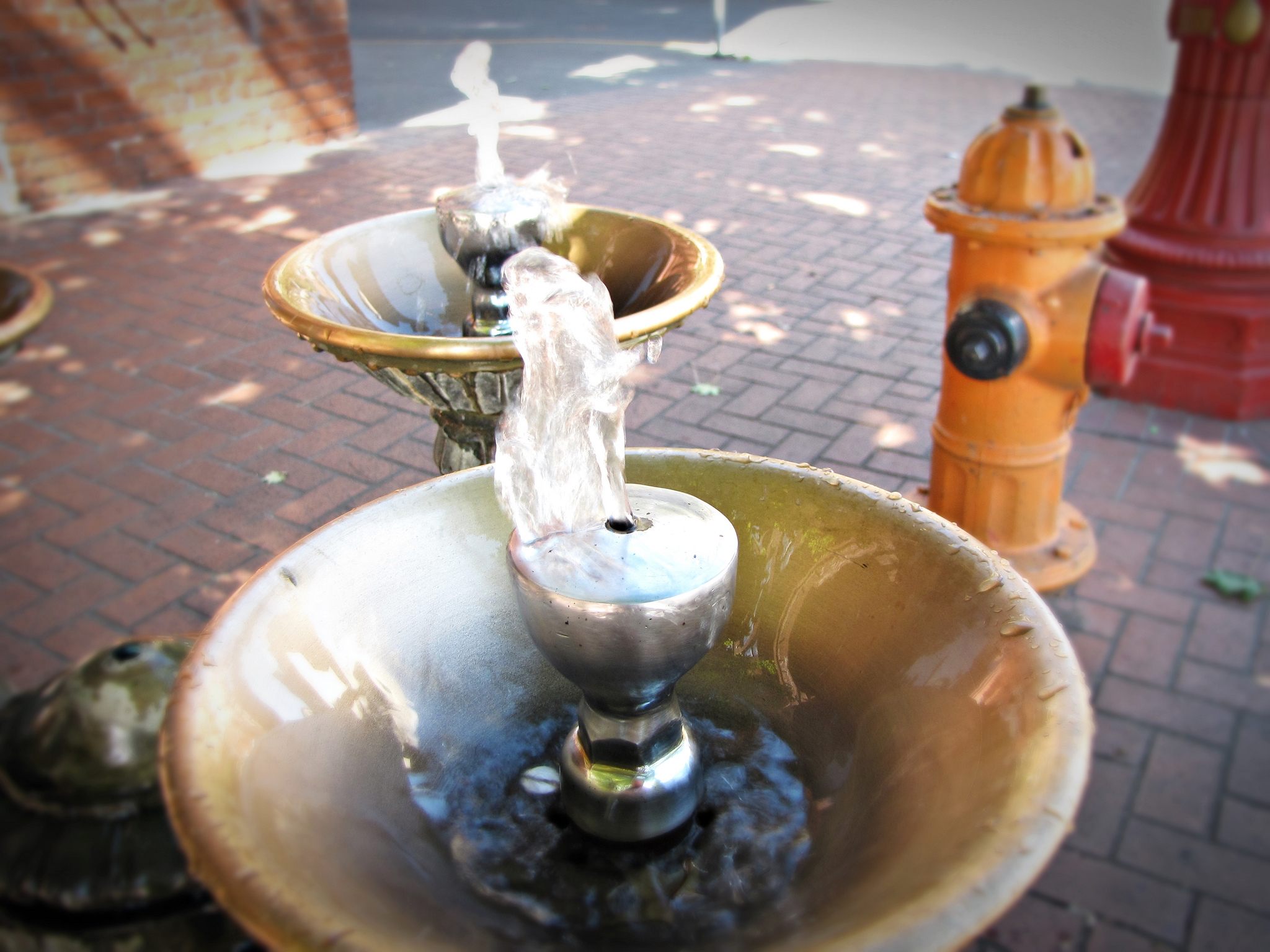The image showcases a close-up of two bowl-shaped water fountains situated outdoors on a sunny day. The nearest fountain is centrally positioned at the bottom half of the image, and a similar fountain is placed directly behind it. Both fountains feature a circular metallic basin with a spout in the middle, from which water sprays upward and then cascades back into the basin in a gentle arc.

To the right of the fountains, there is a prominently visible fire hydrant painted in yellow and red, with a black section toward the viewer that appears to be where a wrench would be applied to operate it. Further back, to the upper right, there is a red, metallic column-like structure, possibly the base of a streetlamp or another outdoor fixture, although its exact purpose is unclear.

The entire scene is set on a dark reddish-brown brick walkway, creating a textured and colorful backdrop. Additionally, in the lower portion of the image, there is a dark, rounded object with multiple layers positioned to the left of the main fountain. In the upper left corner, part of a red brick building is visible, enhancing the outdoor and urban aesthetic of the scene.